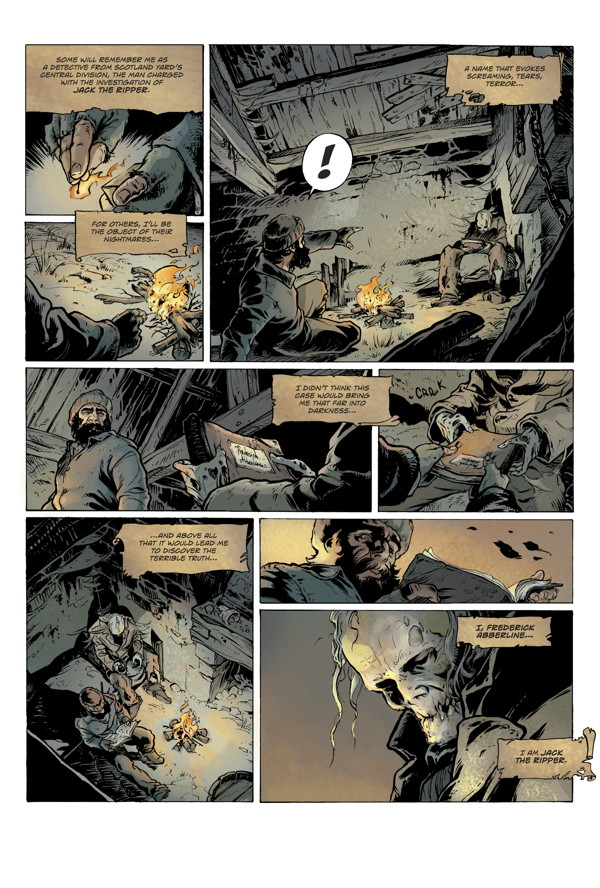The image is a colorful and detailed page from a comic book, displaying nine vertical frames of varying sizes. The page predominantly uses blacks, grayish purples, and oranges to depict a dark setting, likely a cave or abandoned house. In the top frames, a man resembling a sailor with a woollen hat, shaggy black beard, and jumper, is seen lighting a match. The sudden light reveals another character in the corner—an eerie figure with a skull head, lips stitched together, straggly white hair, and tattered clothing. As the sailor investigates, he finds the skull character holding a book, which he then takes to examine. The text, styled like tea-stained beige paper, ultimately reveals a chilling revelation as the skull figure declares, "I am Jack the Ripper."